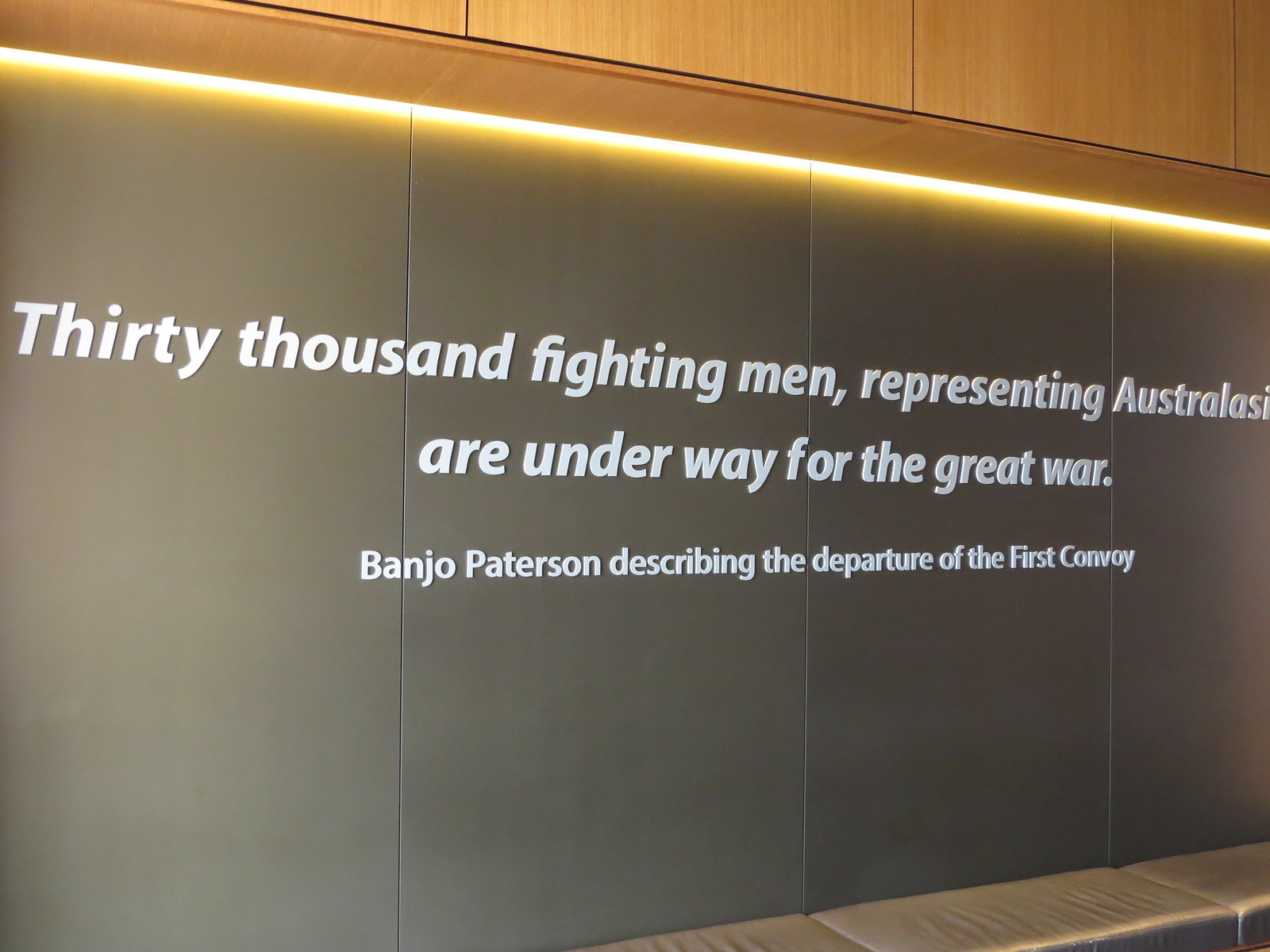The image depicts a slate gray plaque mounted on a wooden framed wall. Above the plaque, wood panels with a brown trim frame the scene, emitting a warm, gold light from underneath, which illuminates the plaque below. The plaque itself is tilted, with its larger portion on the upper left side and tapering towards the right.

The top part of the plaque features a segment of gray wall with white text that reads: "30,000 fighting men representing Australasia are underway for the Great War." Directly below this text, in smaller white print, is a quote attribution: "Banjo Patterson describing the departure of the first convoy." A wooden shelf extends below the gray plaque, completing the framed display.